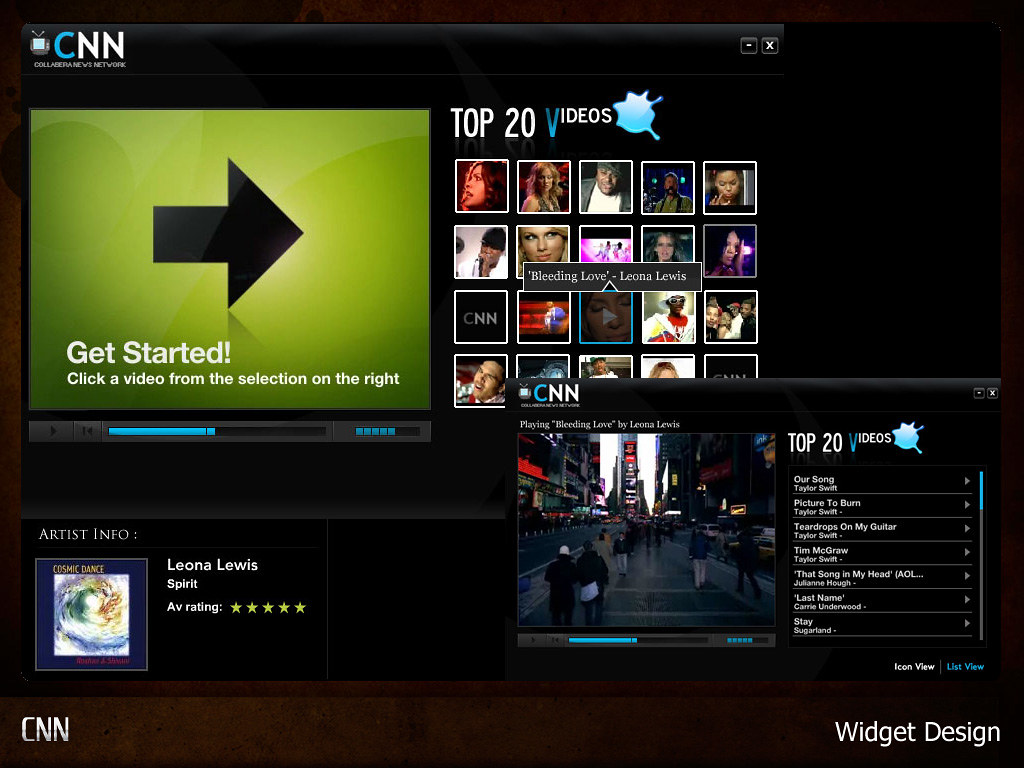The image appears to be a screenshot of a multimedia computer software or website interface with a black background. At the top left, there is a small icon resembling a TV with antennas, displaying the letters "CNN" in uppercase, with the 'C' in blue and the 'NN' in white. Below this, in very small letters, it reads "Collaborative News Network." Adjacent to this on the right is an X and a minus sign icon, likely for window controls. 

Below, there's a green rectangular video player with a large black arrow in the center, accompanied by a "Get Started!" button. Underneath it, text instructs users to "Click a video from selection on the right." To the right of this player is a section labeled "Top 20 Videos," displaying a 5x4 grid of video thumbnails, featuring various singers.

In the bottom left corner, there is artist information for Leona Lewis, showing an album cover with "Spirit" and an AV rating of five stars. Nearby, it mentions "Playing Bleeding Love" with a visual of a cityscape. Both the bottom left and bottom right corners display "CNN" and "Widget TV," respectively. The interface includes a smaller mini player, mirroring the main window but with a scrollable list of songs on the right side, and a blue progress bar at the bottom.